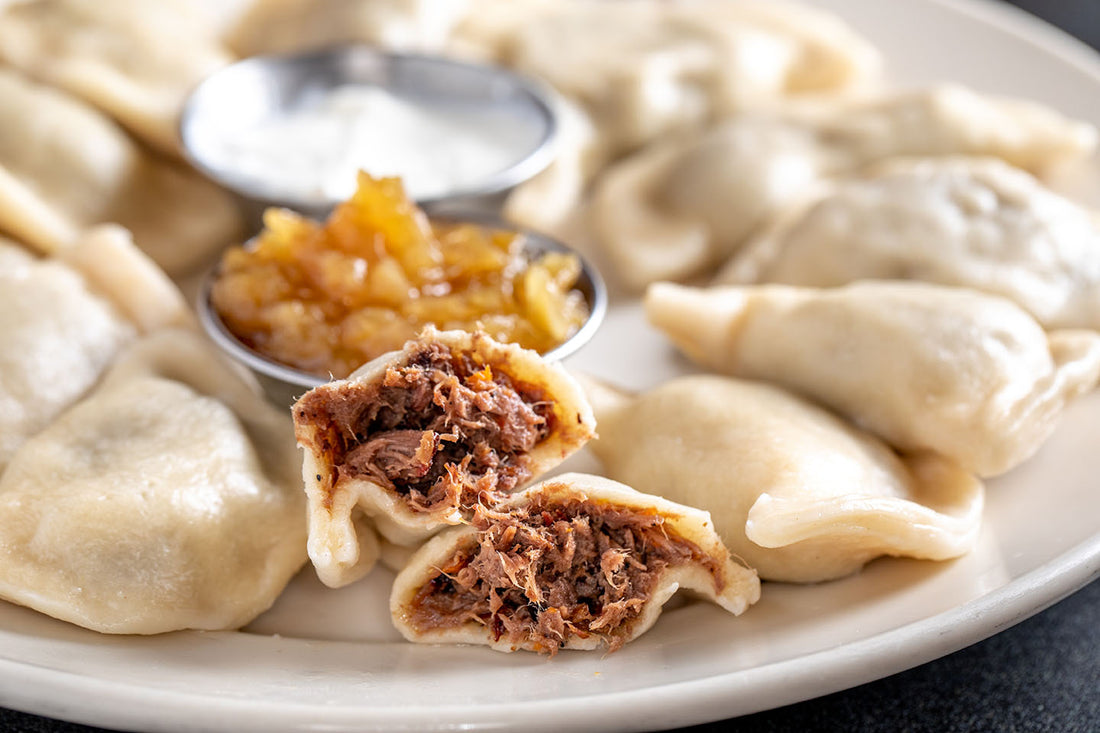This photograph depicts a white circular plate on a black, charcoal-colored countertop, visible only in the bottom corner of the image. The plate is filled with meat dumplings arranged around the edges. One dumpling in the forefront is cut in half, revealing a filling of barbecued beef. At the center of the plate, there are two small circular silver bowls. The front bowl contains a golden, chunky sauce, while the bowl behind it holds a creamy white substance, possibly a sauce or yogurt. The arrangement is visually focused on the halved dumpling, highlighting its meaty interior.